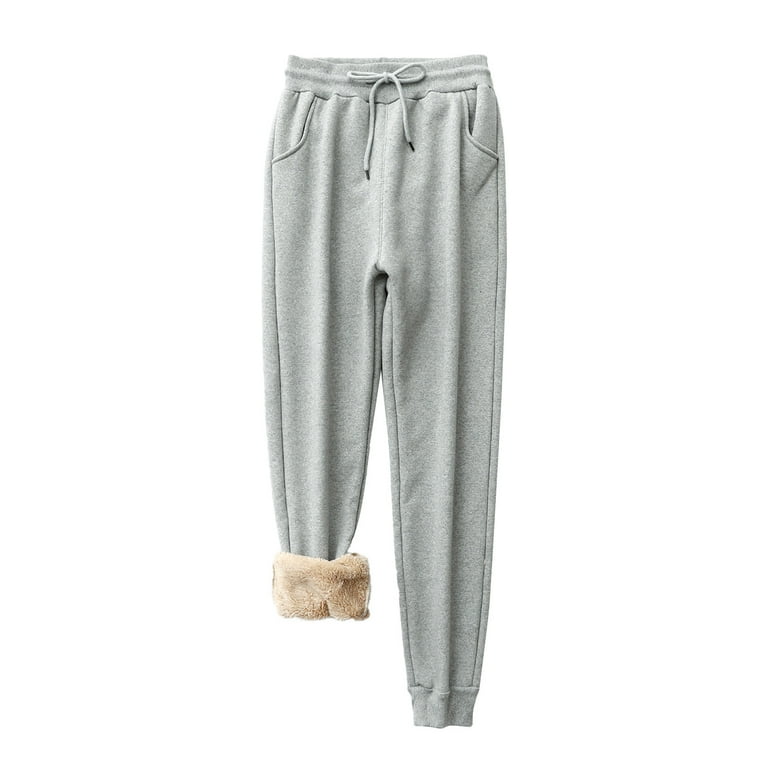This image displays a pair of gray drawstring sweatpants laid flat on a black background, showcasing the front view. The sweatpants feature a waistband with a drawstring tied in a neat bow. Each hip has a pocket, and both legs are meticulously pressed with pleats running their full length. The left pant leg ends with the typical elastic cuff you would expect around the ankle, while the right pant leg is rolled up to just below the knee, revealing a warm, fleece-like, synthetic material in a goldish-brown color that stands out against the otherwise uniform gray fabric. The contrast in the right leg's furry cuff adds a unique touch, making it the only other color in the image. There are no texts or additional colors aside from the gray fabric and the brown of the inside material.